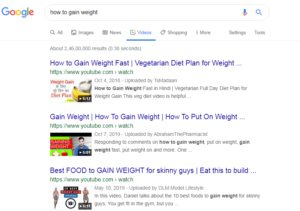**Detailed Image Caption:**
This image is a screenshot of a Google search query for "how to gain weight" displayed in black text within the search bar. In the upper-left corner, the iconic Google logo with colorful capital letters "G-O-O-G-L-E" is visible. Inside the search bar, there is a small microphone icon to the right and a magnifying glass icon signifying the search function. Below the search bar, the typical Google navigation tabs are aligned horizontally, listing categories such as "All," "Images," "News," "Videos," "Shopping," followed by an unreadable blurry section, and then "Settings" and "Tools."

The search results indicate approximately 2.4 billion results for the query. The first search result line reads "How to gain weight fast," followed by a divider line. The second line appears to mention a "vegetarian diet plan for weight." More search result descriptions are partially visible but not entirely legible, with phrases like "gain weight," "how to gain weight," and "how to put on weight." Additionally, the suggestion "best food to gain weight for skinny guys / eat this to build" is partially discernible. The overall image quality is blurry, which impacts the readability of finer details.